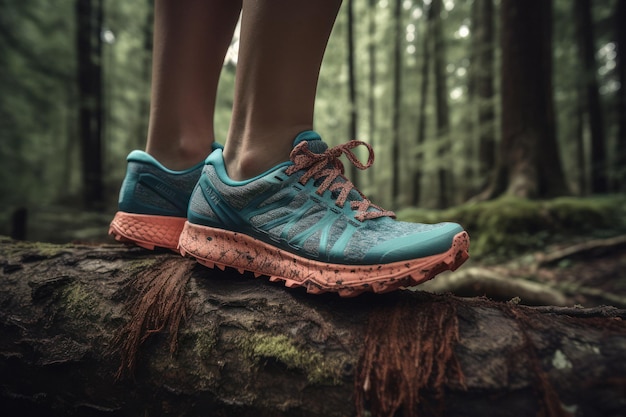The image captures an outdoor scene in a dense, damp forest, with the primary focus on a woman's sneakers standing prominently in the center. The teal-patterned sneakers, accented with gray, boast coral-pink soles and laces speckled with black. The sneakers, worn without socks, suggest casual comfort as the woman stands with her tan legs visible. She is posed on a dark brown tree log covered in patches of green moss, which gives the impression of a rugged terrain. The log itself appears to be nestled in a dirt path, hinting at an adventurous hike. Beyond the tactile focus on the sneakers and log, the background fades into a blur of numerous tree trunks reaching skyward, with diffuse sunlight filtering through the canopy above, enhancing the forest's tranquil yet mysterious ambiance.